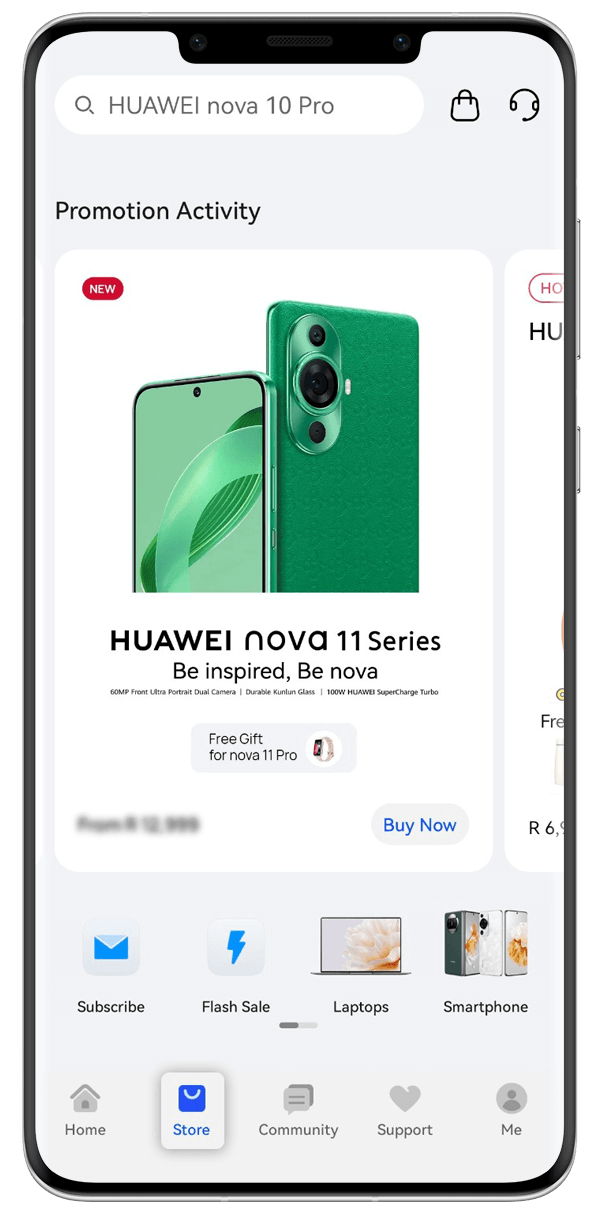The image features a Huawei Nova 10 Pro and Nova 11 Series promotional setup. On the top, there's a speaker and a camera, with the corners highlighting "Huawei Nova 10 Pro." A bag and a phone are visible alongside a headset that mentions "promotion activity." A square overlay reads "The top glass is red thanks to you."

Another phone, which is part of the Huawei Nova 11 Series, displays the slogan "Be Inspired, Be Nova." It boasts a 60 MP front ultra portrait dual camera and mentions having a durable screen backing with a green wallpaper. The rear camera setup is also highlighted.

The promotional content emphasizes "Huawei Supercharged Turbo," offering a free gift for those who subscribe to the Nova 11 Pro. Additional elements include references to flash, a laptop, and a smartphone, suggesting comprehensive tech offerings.

The scene appears to be set in a home-like environment with blue and historic elements, showcasing community support. The edges of the devices are very grey, while the back of the featured phone is white.